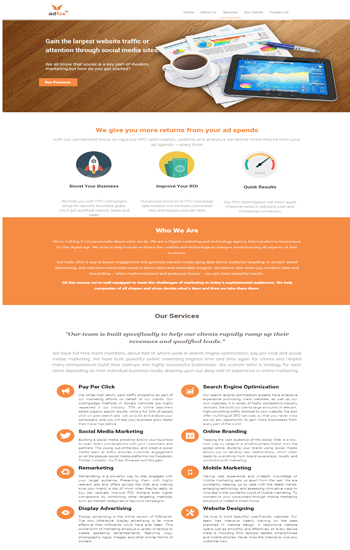The screenshot captures a full view of a website, meticulously trimmed to eliminate the need for a vertical scrollbar, albeit at the cost of readability due to compression. At the very top, a white navigation bar prominently features the logo "AdFox," with several unreadable options in gray font to its right.

Just beneath this navigation bar is a woodgrain-textured rectangle. Within this section, written in white font, are the words: "Gain the largest website traffic or attention through social media sites." Additional white text follows, unreadable due to compression, accompanied by an orange button with similarly illegible white font.

To the right of this primary text block is a cartoonish graphic depicting two sheets of paper on a desk, overlaid with a pen and a tablet. Atop the sheets of paper rests a saucer and cup filled with what appears to be coffee or tea, enhancing the workplace feel of the image.

Further down, a white rectangle contains an impactful message in orange font: "We give you more returns from your ad spends." Beneath this, two lines of black text are present but remain indecipherable.

At the bottom of the screenshot, three horizontally-aligned circles house distinct icons: a rocket ship symbolizing growth or launch, a wad of dollar bills representing financial gains, and a clock indicating time efficiency. These elements collectively illustrate the website's emphasis on maximizing advertising returns and efficiency.